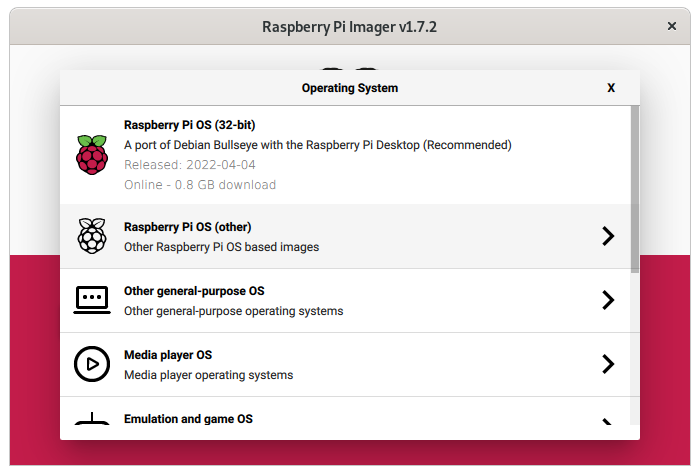The image showcases a computer screen displaying the Raspberry Pi Imager version 1.7.2 interface against a white and pink background. The interface highlights the operating system "Raspberry Pi OS (32-bit)" with additional information indicating support for the Bullseye version with the Raspberry Pi desktop. It is noted as the recommended release, dated April 4, 2022, and is available for online download with a size of 0.8 GB.

Additionally, the interface lists several categories of operating systems available through the Raspberry Pi Imager. These include "Other Raspberry Pi OS based images," "Other general-purpose operating systems," "Media Player OS," and "Emulation and Game OS." To the right of the operating system listings, there is a visible gray scroll bar, indicating that more options are available beyond the initially visible selections.